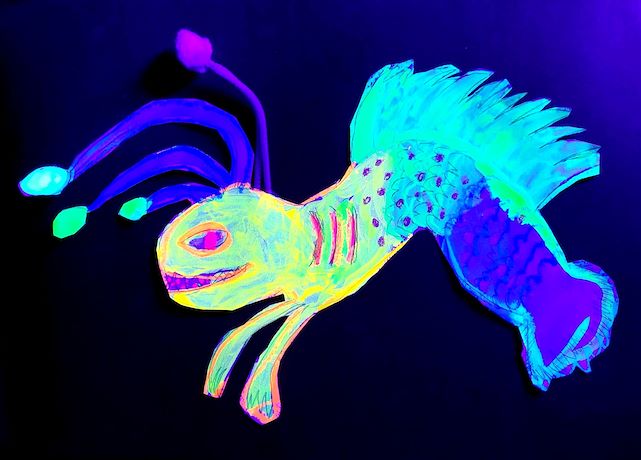This artwork depicts an extraordinary, imaginary creature, reminiscent of a hybrid between a fish and a four-legged animal, perhaps even evoking images of an anglerfish with its unique features. The background transitions from dark black at the bottom to a deep blue at the top, creating a dynamic and captivating backdrop. The creature itself boasts a stunningly vibrant palette. 

Its head is lizard-like, painted a green hue with splashes of yellow and orange, leading to a predominantly purple mouth filled with sharp, hot pink teeth. One striking eye glows hot pink, accented with greenish-yellow and orange eyelids. Emerging from its crown are four antennae-like tentacles, predominantly dark blue with purple accents, each ending in distinct circles - the longest featuring cyan blue with white dots, while the other two maintain a green with blue highlights.

The creature’s torso begins as yellowish-green with orange accents, adorned with three maroon claw-mark-like lines that transition into cyan blue towards the lower body. This section is speckled with aligned purple dots, continuing down to its legs. These legs are elaborately painted with wavy dark blue and purple stripes, with blue outlines in the front and a gradient from green to bluish-green towards the rear. Notably, cyan-green feathers or spikes sprout a quarter of the way down the back legs.

The creature’s physical appearance concludes with features reminiscent of fins and tentacles, painting a jarring picture of a fish-like being, yet possessing attributes of a terrestrial animal. Its dorsal section showcases shades of light and dark blue, while the torso and front fins exhibit a radiant neon blend of yellow, pink, and purple. The overall effect is a hyper-neon, surreal creature, seemingly the imaginative work of a young artist, displaying intricate polka dots in its midsection.